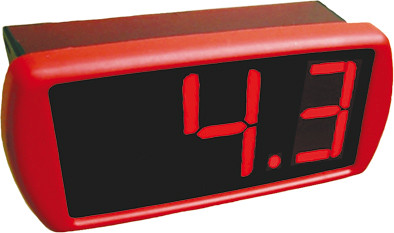The image depicts a rectangular electronic device with a digital readout. The device has a red border surrounding a black background where the digital numbers are displayed. The numbers themselves are shown in red. The device is tilted, appearing as if the left side is lower than the right, creating a diagonal orientation. The digital display shows the number "4.3." The digit "4" is constructed from red LED segments forming a pattern of a vertical line descending, a horizontal line across the middle, and another vertical line descending on the right, while the digit "3" is made up of curved and straight red LED segments with a noticeable gap between the upper and lower halves.